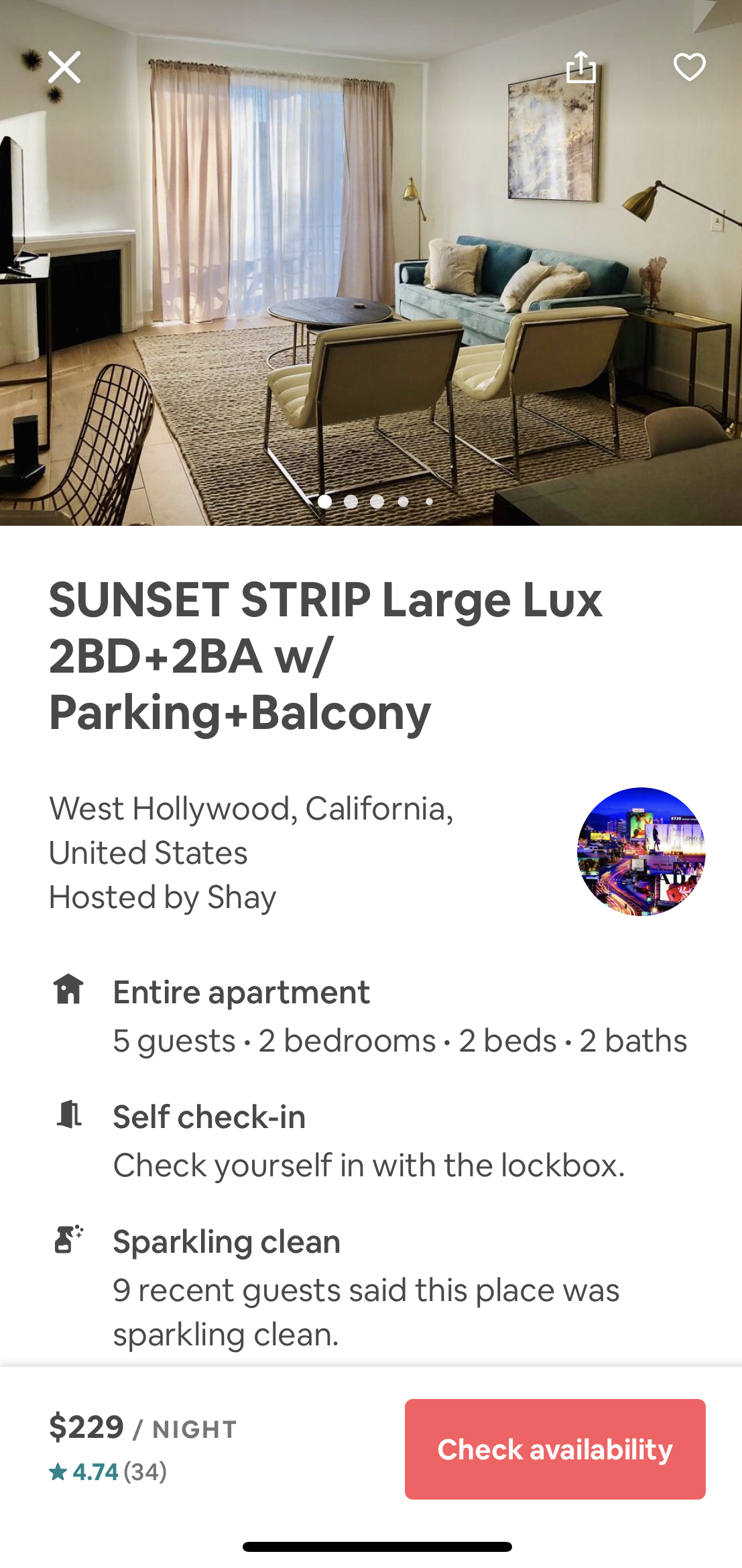This image is a mobile screenshot taken on an iPhone, identifiable by the distinct bottom bar that lets users exit the app. The screenshot showcases a home listing, likely from a platform such as Airbnb. At the top of the screen, there are several icons: an 'X' for exiting the page, a share icon depicted as an arrow emerging from a square, and a heart icon indicating the item has been favorited.

The main section of the screenshot displays a high-resolution image of what looks to be someone's living room. Visible in the room are several windows, a couch, some chairs, a television, and a desk, suggesting a comfortable and well-furnished space. Accompanying this image are at least five smaller pictures, providing a comprehensive view of the property.

This listing is for a "One Strip, Large, Luxe, Two Bedroom, Two Bath Apartment with Parking and Balcony" located in West Hollywood, California, United States. It is hosted by someone named Shea. The entire apartment is available and can accommodate up to five guests with its two bedrooms, two beds, and two bathrooms. The listing emphasizes convenience with self check-in through a lockbox. Additionally, the property is praised for its cleanliness, as noted by nine recent guests who described it as "sparkling clean."

The price for staying at this apartment is $229 per night. It boasts a high rating of 4.74 stars, based on 34 reviews. A "Check Availability" button is prominently featured, inviting potential guests to book their stay.